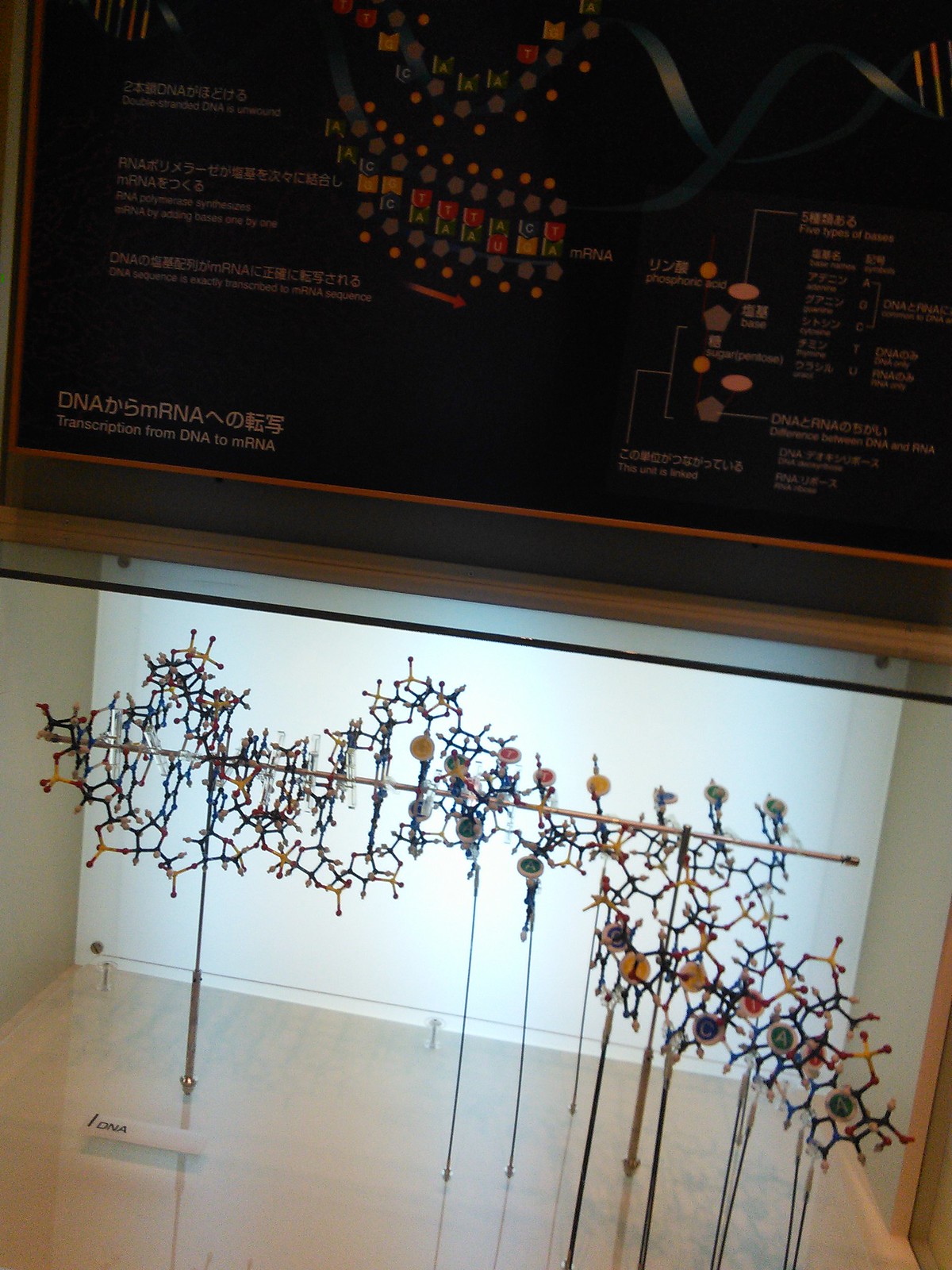This detailed image depicts a museum exhibit focused on the biological processes involving DNA and mRNA. At the top of the image, there is a poster with a black background, featuring detailed diagrams and multi-colored illustrations (green, red, yellow, and blue) that explain the transcription process from DNA to mRNA. Although most of the text on the poster is in a different language and unreadable, key terms like "DNA" and "mRNA" are discernible.

The bottom section of the image showcases a series of artistically designed 3D models representing DNA and mRNA. These models are carefully enclosed behind a glass case, resting on a wooden surface. The colors of the models correspond with the colors used in the diagrams above. Additionally, a small tag within the glass case is labeled "DNA." The entire scene, captured indoors from an angled perspective, gives the impression of a cohesive educational display found in a museum setting. The various colors observed in the exhibit include brown, black, gray, orange, red, green, and silver, adding vibrancy to the detailed and informative setup.